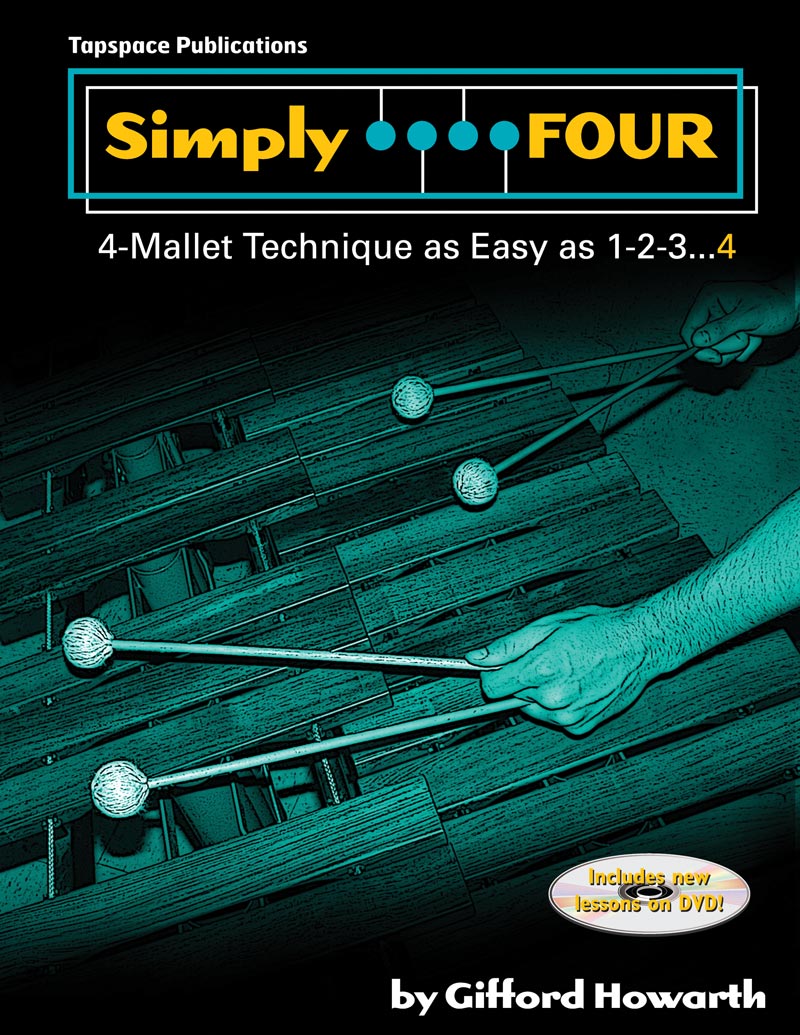The front cover of the instructional guide is vibrantly colored and features detailed branding and imagery centered around the theme of four mallet percussion. At the very top left, on a black background, white text reads "Tap Space Publications." Centrally positioned at the top is the title, "Simply Four," with the word "Simply" and the number "4" distinctly separated. Beneath this title, the subtitle reads, "4-Mallet Technique, as easy as 1-2-3...4," with the final "4" in a bold yellow. Prominently featured in the middle of the cover, a pair of hands skillfully holds four mallets above a xylophone, illustrating the technique discussed in the book. A graphical representation of the four mallets, alternating in blue and white with blue circles at the ends, is situated between "Simply" and "4." The background predominantly showcases a gradient tint that fades from teal blue to a lighter hue. On the bottom right, author credit appears in white text, stating "By Gifford Howarth." Additionally, a reflective CD icon with a rainbow sheen is located here, containing yellow text that enthusiastically announces, "Includes new lessons on DVD!" Overall, the cover merges instructional clarity with compelling visuals, creating an inviting introduction to four mallet percussion techniques.